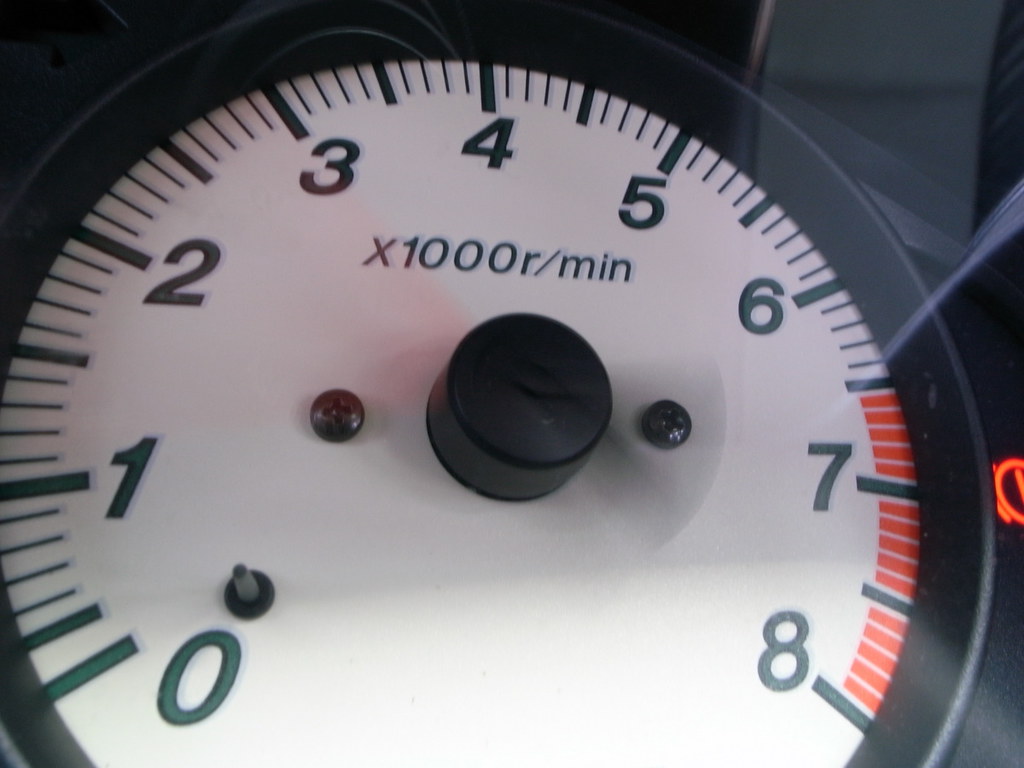This close-up image captures the RPM gauge of a high-performance sports car. The gauge features a white background with black numerical markings and increments, providing clear readability. Prominently displayed at the top center of the gauge are the words "x1000 R/min," indicating the revolutions per minute in thousands. To the right, there is a red icon, the purpose of which is unclear, possibly serving as a warning light. Notably, the red zone on the gauge starts from 6,500 RPM and extends to 8,000 RPM, suggesting that exceeding this range pushes the engine into its maximum performance threshold. Although the gauge is not currently visible, there is a faint presence of the needle, implying that the engine is running and the vehicle is in motion. The gauge's center is black, adding to its sleek design. The photo appears to be taken through a glass pane, as evidenced by the slight reflections obstructing a clear view, and a check engine light is faintly visible off to the right. The image seems to be captured by positioning the camera within the car's dashboard area, focusing exclusively on the RPM gauge.